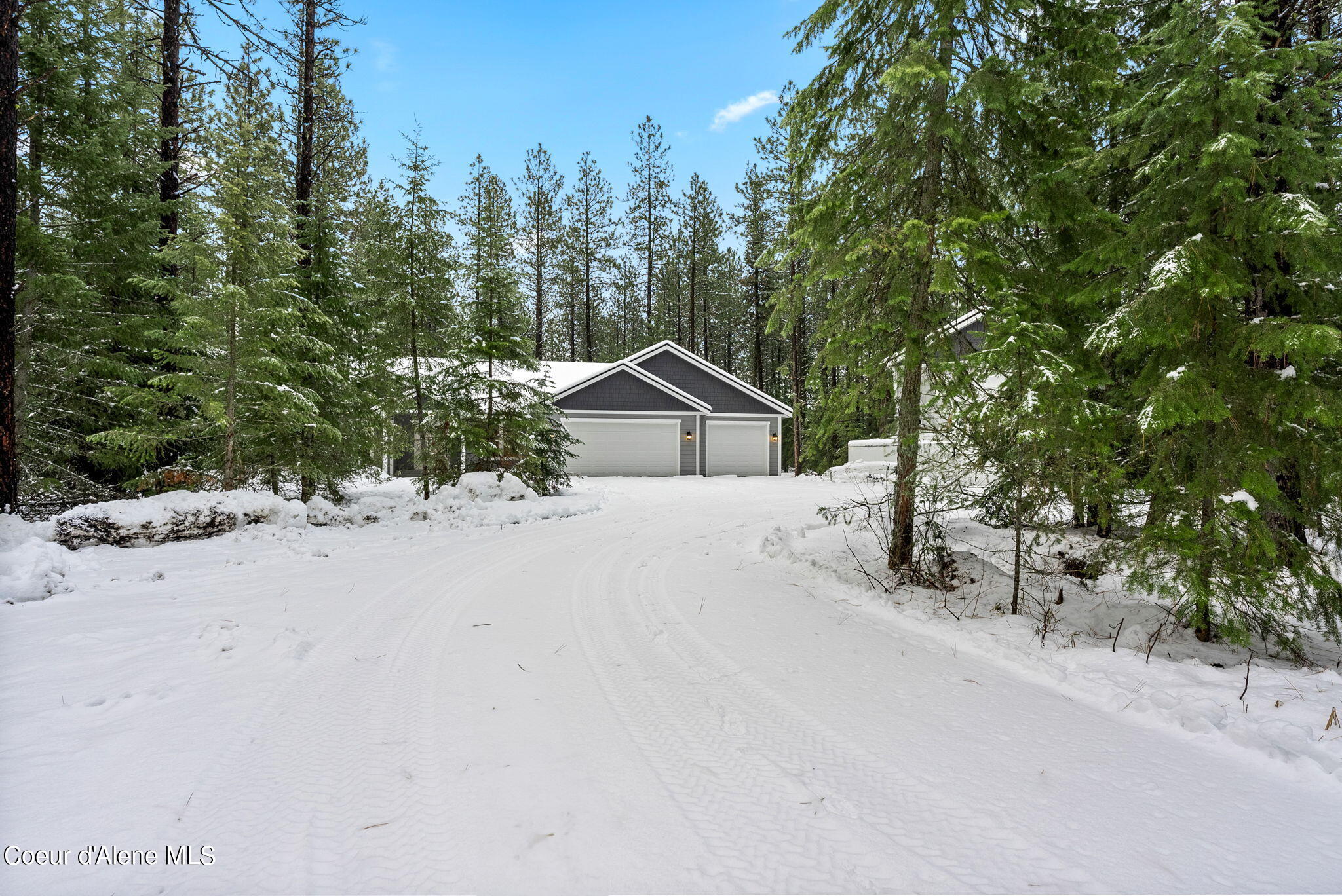The image depicts a high-quality photograph of a small house set amidst a snowy, wooded landscape, viewed from the road in front. The house features a three-car garage with white doors, positioned in a graduated form—one large door at the front and a smaller one to the right. Beside each garage door, there are outdoor lamps that are turned on despite the daylight, casting a warm glow. The driveway, covered in a pristine layer of snow and etched with tire tracks, is broad, wide enough to fit four cars side-by-side and stretches long, meandering up to approximately 100 yards towards the house, forming an S-shape. 

Flanking the driveway, tall fir and pine trees, some lightly dusted with snow, add to the serene winter scene while the trees in the backdrop remain mostly green with occasional bare branches. The house itself, with a sharply peaked roof partially coated in snow, has a dark blue facade section beneath the peak and white columns lining the front portico. The sky above is a clear blue, punctuated by a few small, white clouds, enhancing the winter tranquility of the scene. The photograph appears to be part of a real estate listing, indicated by the label "Sir Delene MLS."